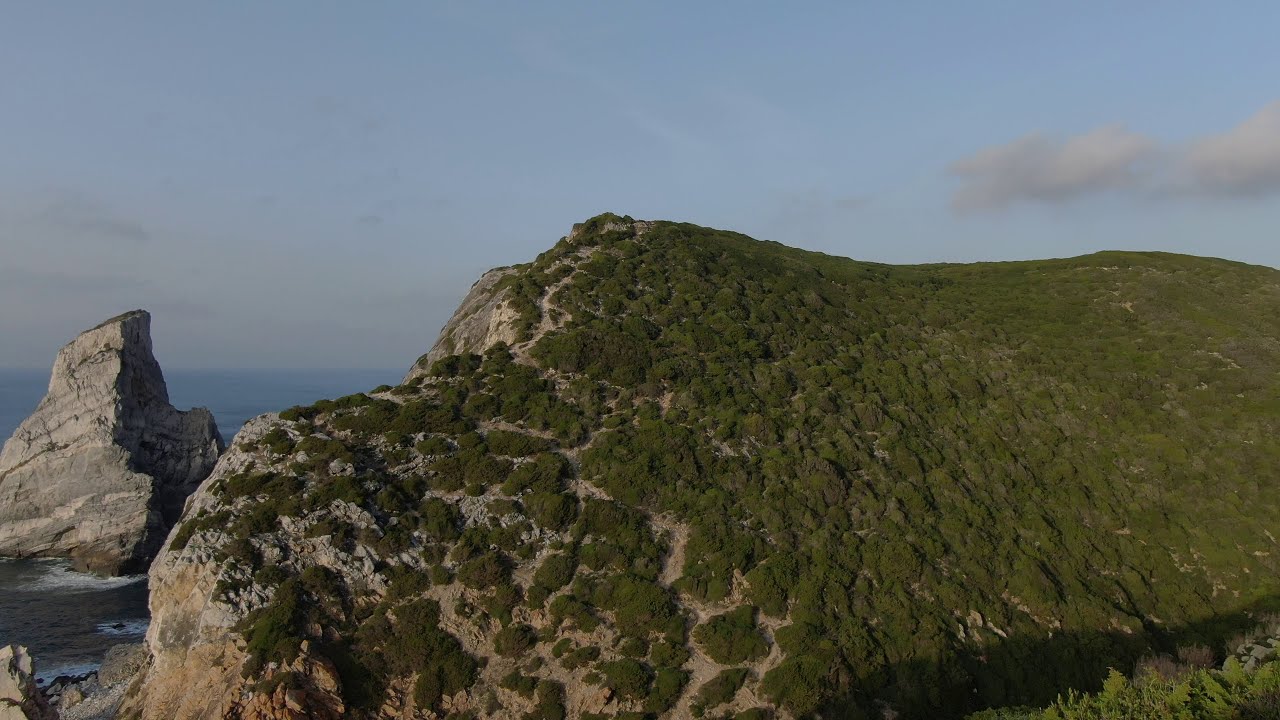The image captures a rugged cliffside that spans nearly the entire width of the frame, from right to almost the left edge. The cliff appears as a rock-heavy hill and is covered with vivid green patches of moss, particularly dense towards the top and more interspersed with rocks and dirt to the left. The rocks, predominantly grey, extend into the ocean, meeting dark blue waters. To the left side, a distinct rock structure juts out from the water, displaying strata of dark and light grey hues. The ocean between the cliff and the rock structure also carries the dark blue of the distance. Above, a light blue sky with scattered small white clouds adds a gentle, airy ambiance to the scene. There are shadowy gullies and hints of complex rock formations that add an extra layer of rugged texture. The cliff, with its tree-covered sections displaying a bird-like shape when viewed from above, has dense foliage that opens up to reveal more earth tones on the left.